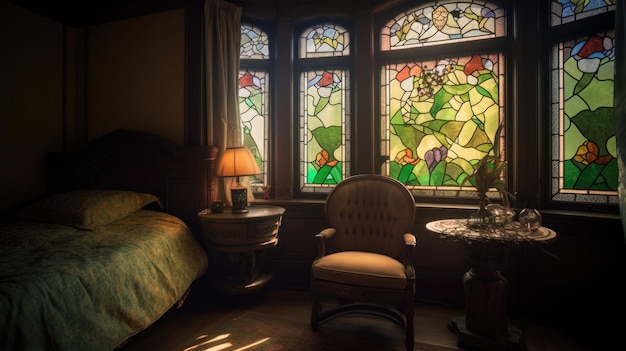The photograph captures an indoor scene of a vintage bedroom bathed in a dim, ambient light. The room exudes an early 20th century or late 19th century Art Deco aesthetic, characterized by its dark, wooden decor and intricate stained glass windows. On the left side of the room is a bed adorned with a floral-patterned blanket in blue and white, complete with a matching pillow and a robust wooden headboard. Adjacent to the bed, a circular wooden nightstand holds a lit lamp with a dark yellow shade, casting a warm glow that highlights the room’s features.

At the center of the image, a plush tan chair with wooden arms and legs stands next to another circular wooden table, emphasizing the consistent usage of wood throughout the space. Behind the chair and on the right side of the bed, the room is graced by a series of four arched stained glass windows, each framed in wood. These windows are a focal point, boasting designs of green leaves outlined in black veins, with splashes of light blue, beige, pink, and red adding a delicate beauty to the otherwise dark environment. The wooden floors and the white walls further contribute to the room's classic and slightly luxurious feel, making it appear reminiscent of a speakeasy from a bygone era.